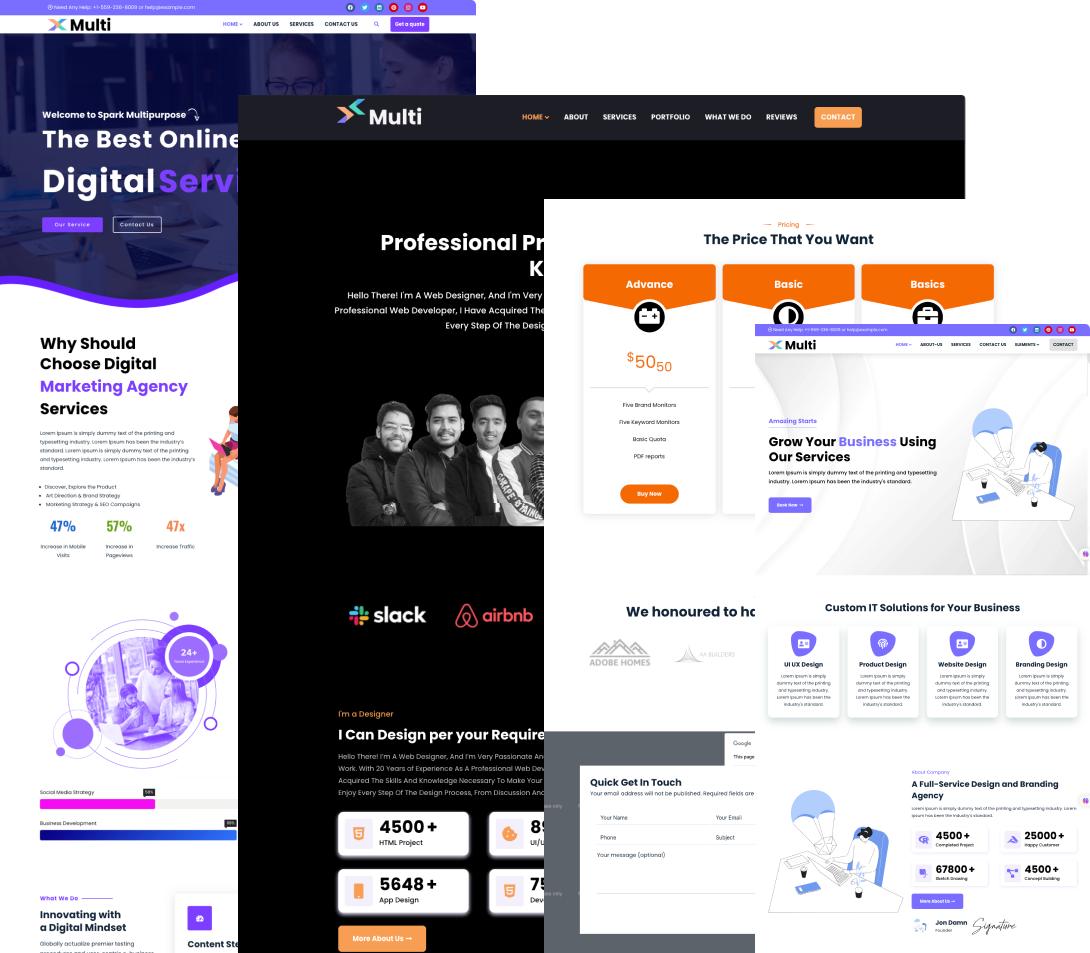The image depicts a series of four overlaid browser tabs, each presenting different sections of what appears to be the same website and gradually decreasing in size from left to right.

1. **Farthest Back Tab (Largest) on the Left:**
   - **Title:** Multi
   - **Description:** "The best online digital services."
   - **Content:** Features an article titled "Why you should choose digital marketing agency services," accompanied by graphs and additional text.
   - **Color Scheme:** Predominantly purple and white.

2. **Second Tab to the Right:**
   - **Title:** Multi
   - **Navigation Menu:** Includes options for Home, About, Services, Portfolio, What We Do, Events, and a Contact button.
   - **Main Content:** A partially visible text at the top, obscured by the page in front of it, and a picture of people below the menu. 
   - **Additional Details:** Buttons for Slack and Airbnb, and text stating "I'm a designer. I can design per your required [something]." Includes buttons for HTML projects and app design.
   - **Color Scheme:** Black background.

3. **Third Tab to the Right:**
   - **Title:** Multi
   - **Section Title:** "The price that you want."
   - **Pricing Plans:** Three tabs labeled Advanced, Basic, and Basics. The Advanced plan on the far left lists a price of 50-50.
   - **Feature:** A "Quick get in touch" form at the bottom.
   - **Color Scheme:** Not explicitly mentioned.

4. **Farthest Right Tab (Smallest):**
   - **Title:** Multi
   - **Headline:** "Grow your business using our services."
   - **Font:** Too small to read clearly.
   - **Color Scheme:** Similar purple and white theme as the farthest left tab.

Overall, the four tabs showcase different aspects of a website related to digital marketing services, with a coherent but varied design presentation.